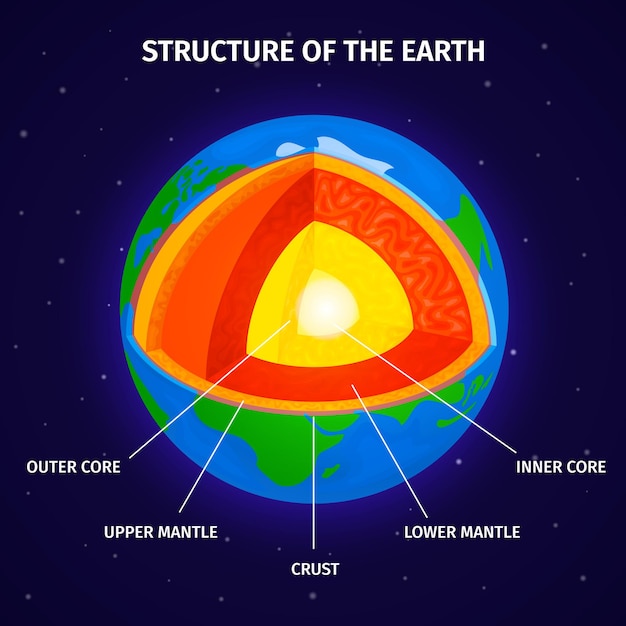The image showcases a detailed, educational poster titled "Structure of the Earth," set against a deep blue, starry background with white dots representing stars. At the center of the poster is a simplified, cross-sectional depiction of the Earth, cut away to reveal its internal layers. The outermost layer is the **crust**, which features land and water surfaces. Just beneath the crust is the **upper mantle**, depicted in an orange-yellow hue. Below that is the **lower mantle**, represented by a thick, bright red layer. Following the lower mantle is the **outer core**, which is a vivid bright yellow. At the very center lies the **inner core**, illustrated as a bright white sphere. Each layer is clearly labeled in white text, emphasizing the structure of the Earth from the crust down to the inner core. The entire visual is both colorful and informative, set in the middle of a night sky backdrop to enhance its educational appeal.